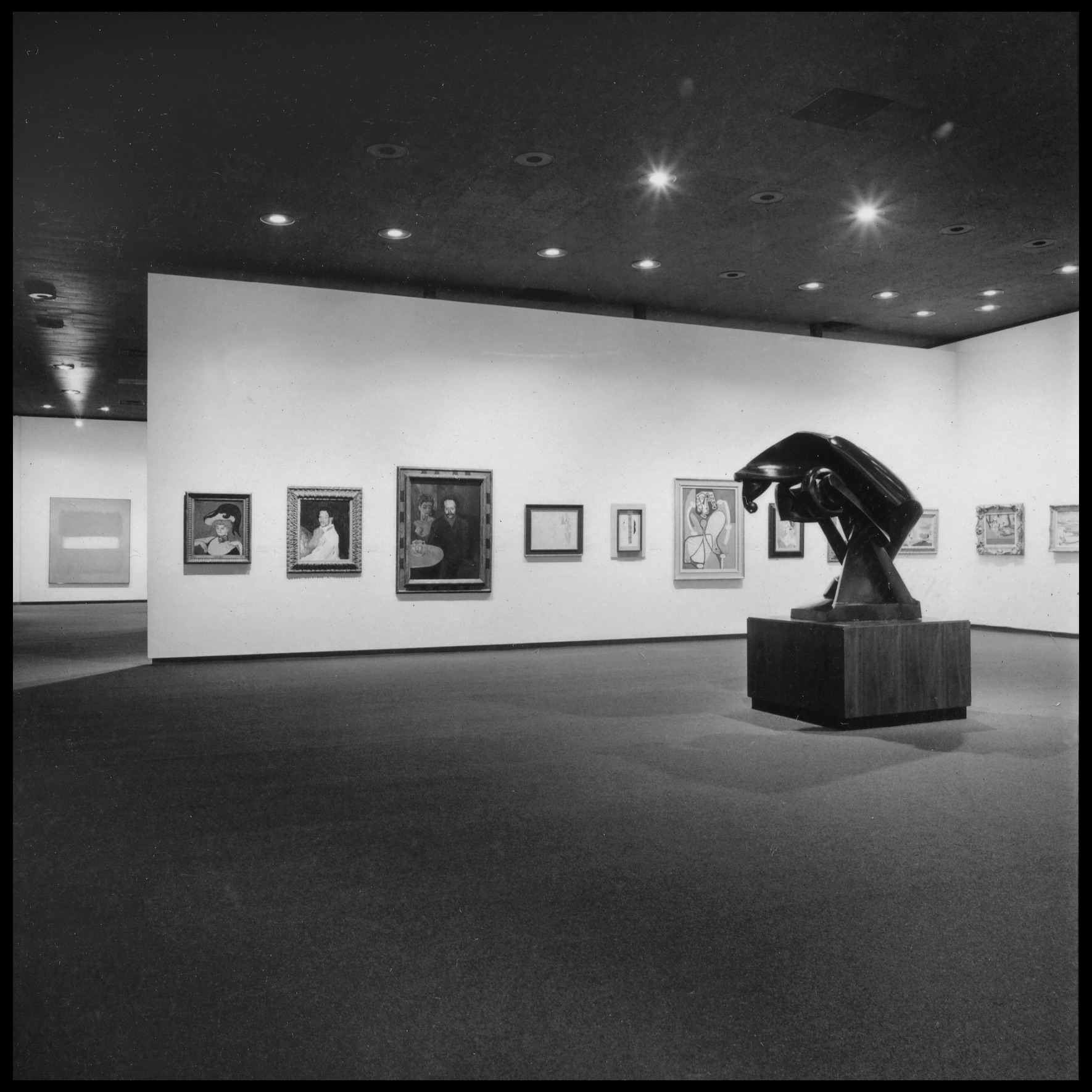This square, black and white photograph depicts a dimly lit art gallery featuring a central, abstract modern art sculpture resting on a substantial square display stand. The gallery showcases walls adorned with a variety of framed artworks, including both abstract pieces and portraits. Approximately eight to nine framed pieces of varying sizes can be seen, with one notable larger portrait featuring a male and female, alongside another large, indistinct geometric abstract piece. The image, taken from a distance, captures the spaciousness of the gallery and hints at an additional pathway leading to another display area. The room is minimally illuminated by ceiling lights, highlighting the contrast between the white walls and the presumed gray carpeting.